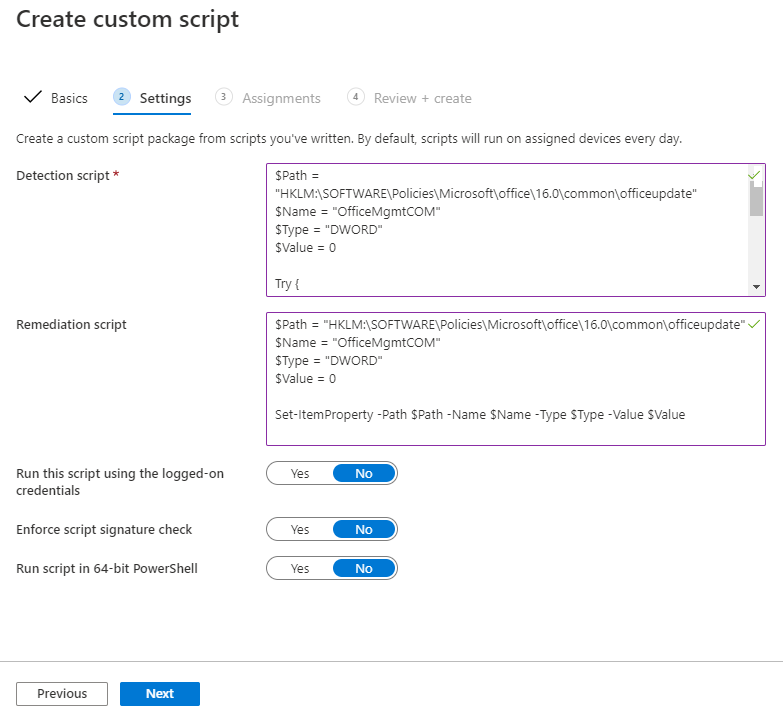In the top left corner, there is an option labeled "Create Custom Script." Following this downwards is a check mark next to "Basic" and then a number "2" within a blue circle labeled "Settings," which is underlined. Beneath this, it mentions "Three Assignments for Review" followed by the "Create" option.

Further below, it reads: "Create a custom script package from scripts you've written. By default, scripts will run on assigned devices every day." The term "detection script" is stated, followed by "REMediation scripts" spelled with spaced-out letters. Additionally, there is an option "Run this script using logon credentials," with Yes and No choices available, where "No" is highlighted.

Next, there's a box for "Enforce script signature checks" with Yes and No options, where "No" is checked. Another option is "Run script in 64-bit PowerShell," also presenting Yes and No choices, where "No" is highlighted.

At the bottom of the interface, you can find "Previous" and "Next" buttons. There is also a script section displaying code snippets such as "path =" or "name = officeMgmtCOM" or "type = word" or "value = 0."